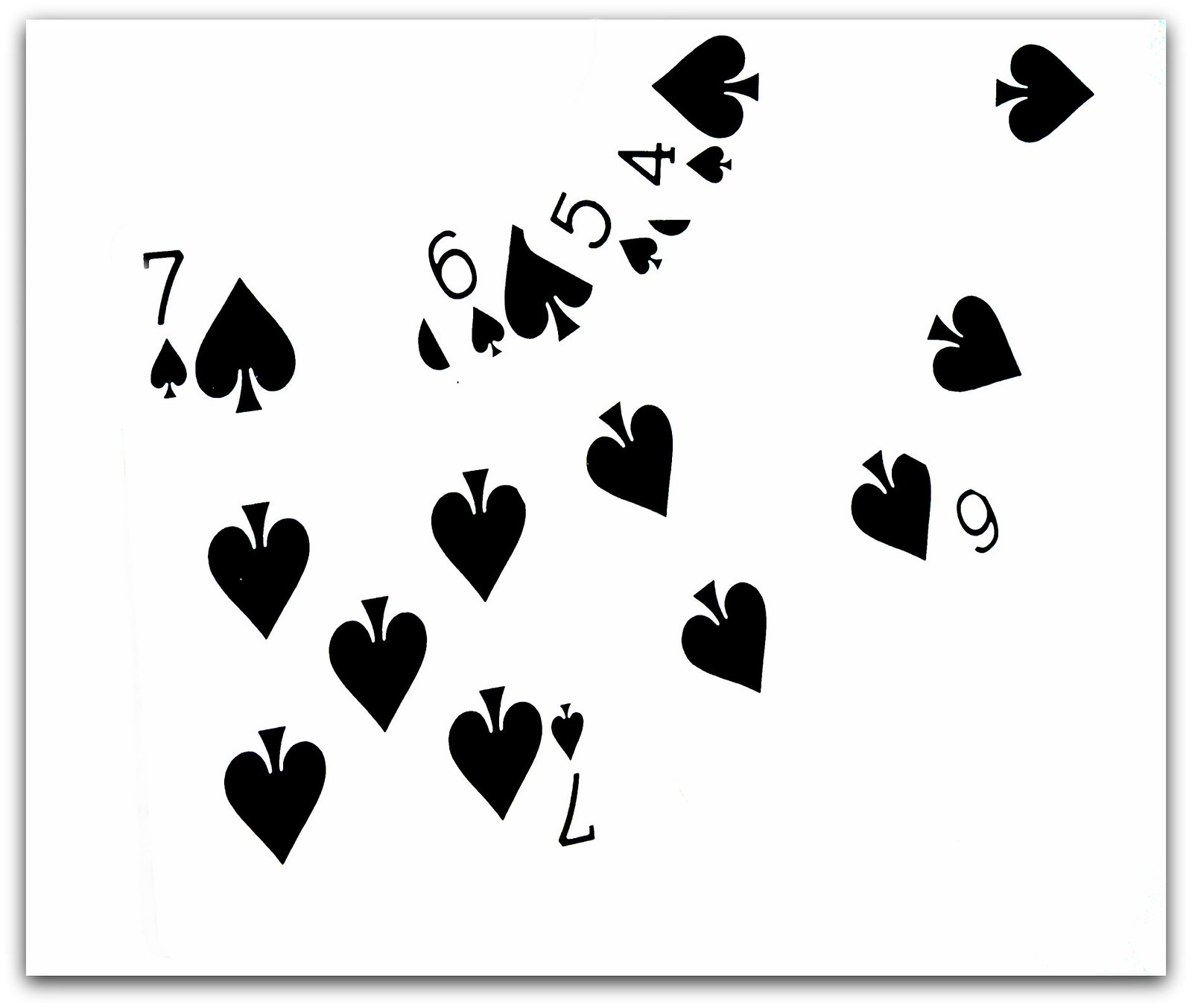This image features a computer-generated, clip art style depiction of a series of four white playing cards, each with the black club suit. The cards appear to be almost layered or photocopied over a larger white rectangle, partially obscuring each other. The overlapping effect results in parts of each card being cut off, creating an incomplete visual of the cards' faces. 

The rectangular background is predominantly white with sharply defined gray borders, and its dimensions indicate a width greater than its height, with an approximate width-to-height ratio of 60:40. Within this background, the four playing cards are arranged in a somewhat haphazard stack, starting from the bottom left with a Seven of Spades. Above it, at a slight angle, is a Six of Spades, followed by a more sharply angled Five of Spades, which is nearly hidden by the topmost card, a Four of Spades. 

The majority of the spade symbols on the cards are oriented pointing downwards, except for those on the top edges of the Seven, Six, Five, and Four of Spades, contributing to the overall layered and overlapping appearance of the image.